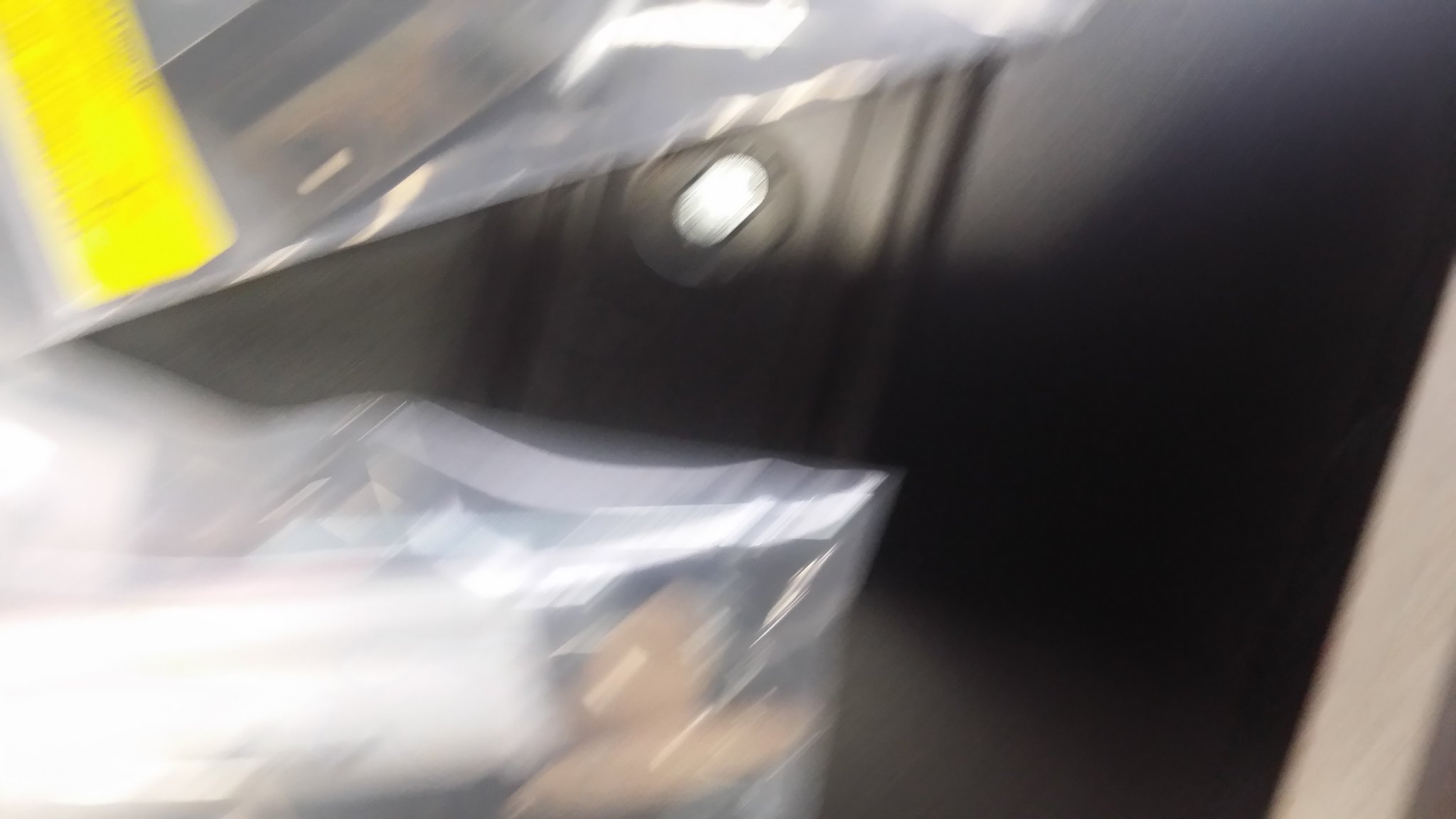The image is heavily blurred, making it difficult to discern specific details. The background, which appears to be black, could be a door, wall, cupboard, or some other fixture, positioned at an angle that obscures clear identification. In the foreground, the edges of several plastic bags are visible. The most prominent bag is centrally located with its corner extending off the frame towards the lower left-hand side. Additionally, the upper left-hand corner of the image shows another plastic bag, which contains a yellow ruler. About one to two inches of this ruler are visible, adding a splash of bright color to the otherwise dark and indistinct scene.